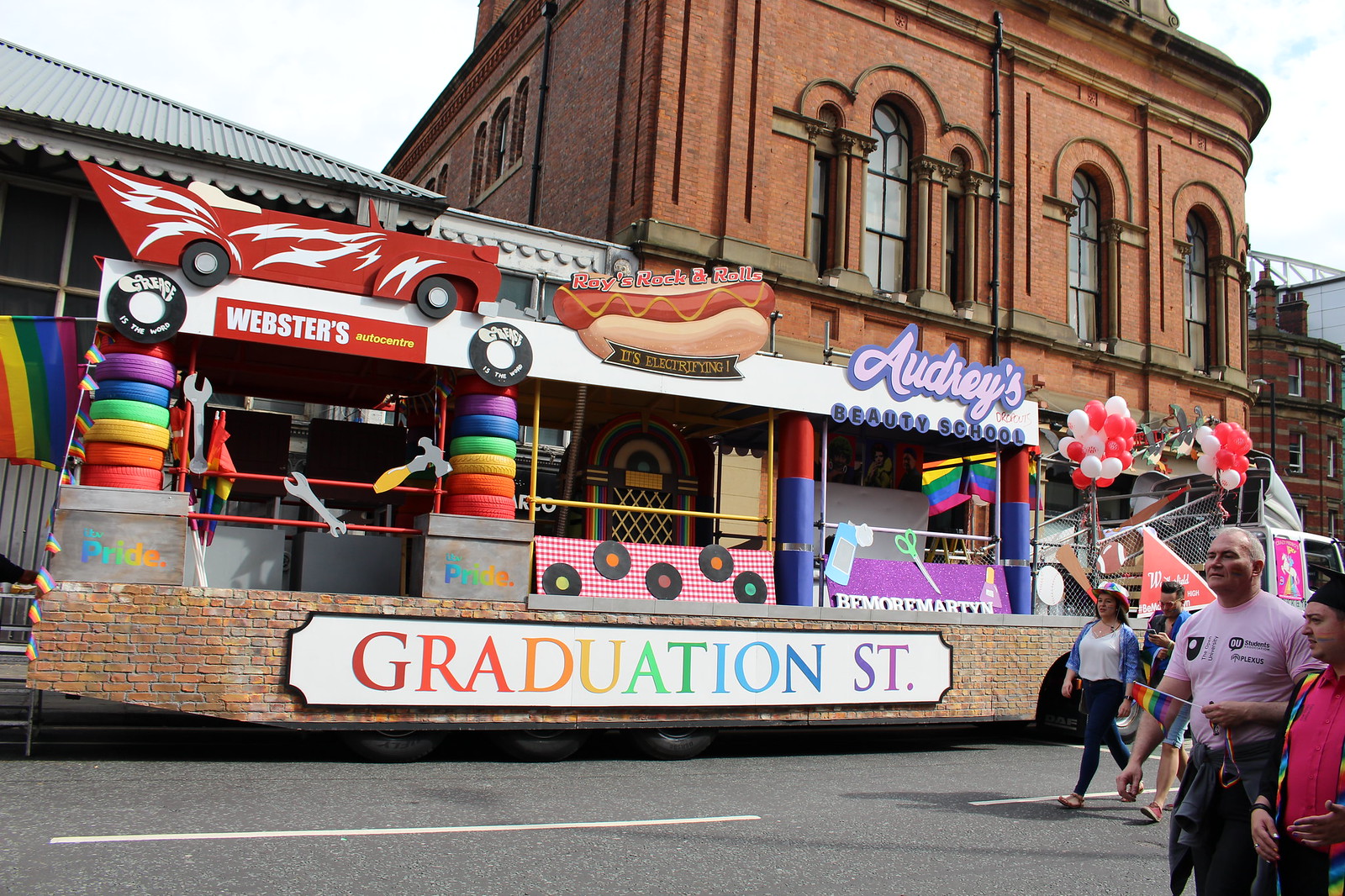The image showcases a colorful parade underway on a blacktop street, featuring a lively Pride float celebrating Graduation Street. Prominently displayed in rainbow text on a white sign, the float is designed with a base resembling a red brick floor. It includes several themed sections separated by poles. On one side is Webster's Auto Center, characterized by rainbow-colored tires, wrenches, hammers, and an old-fashioned red wooden car adorned with white lightning bolts. The center of the float resembles a 1950s diner with a jukebox embellished with rainbows and a hot dog sign above it, labeled Roy's Rock and Rolls. On the opposite end, Audrey's Beauty School is marked by a rainbow flag and text. In the background, two tall brick buildings with ornate, cathedral-like windows rise against a sky filled with white clouds. Numerous bystanders, including a man in a light pink shirt and a woman in a white shirt, black leggings, and a ball cap, are visible. Additionally, red and white balloons further enhance the celebratory atmosphere of the scene.